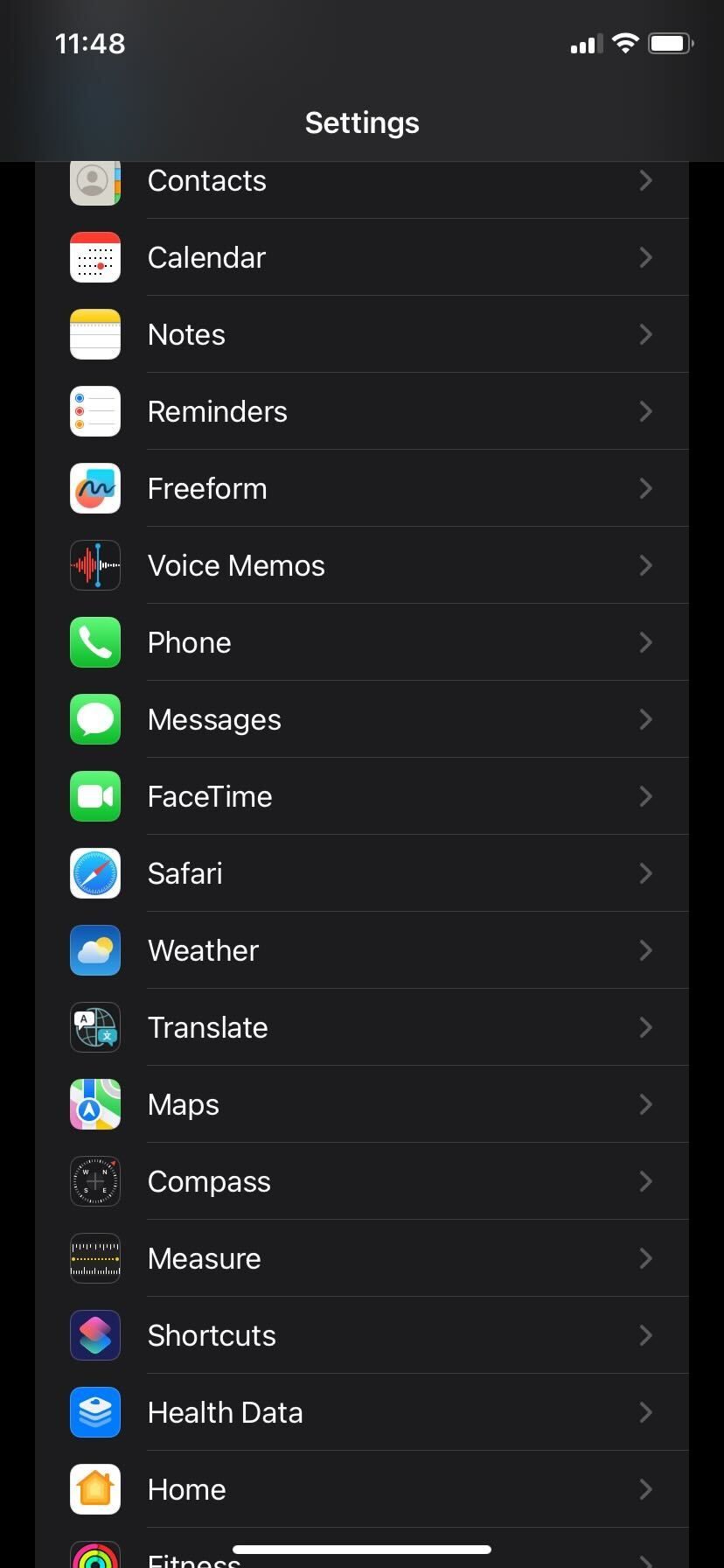This screenshot displays the settings interface of a device. The top of the screen features standard power options. The background is entirely black with subtle grey lines separating each item. On the right side of the screen, arrows indicate the ability to navigate further. Centrally positioned is the heading "Settings," written in white with each word capitalized. Below this, in a white font, are several standard application labels accompanied by their respective icons. These include: Contacts, Calendar, Notes, Reminders, Freeform, Voice Memos, Phone, Messages, FaceTime, Safari, Weather, Translate, Maps, Compass, Measure, Shortcuts, Health Data, and Home. The screen allows for scrolling to reveal additional items in the list.